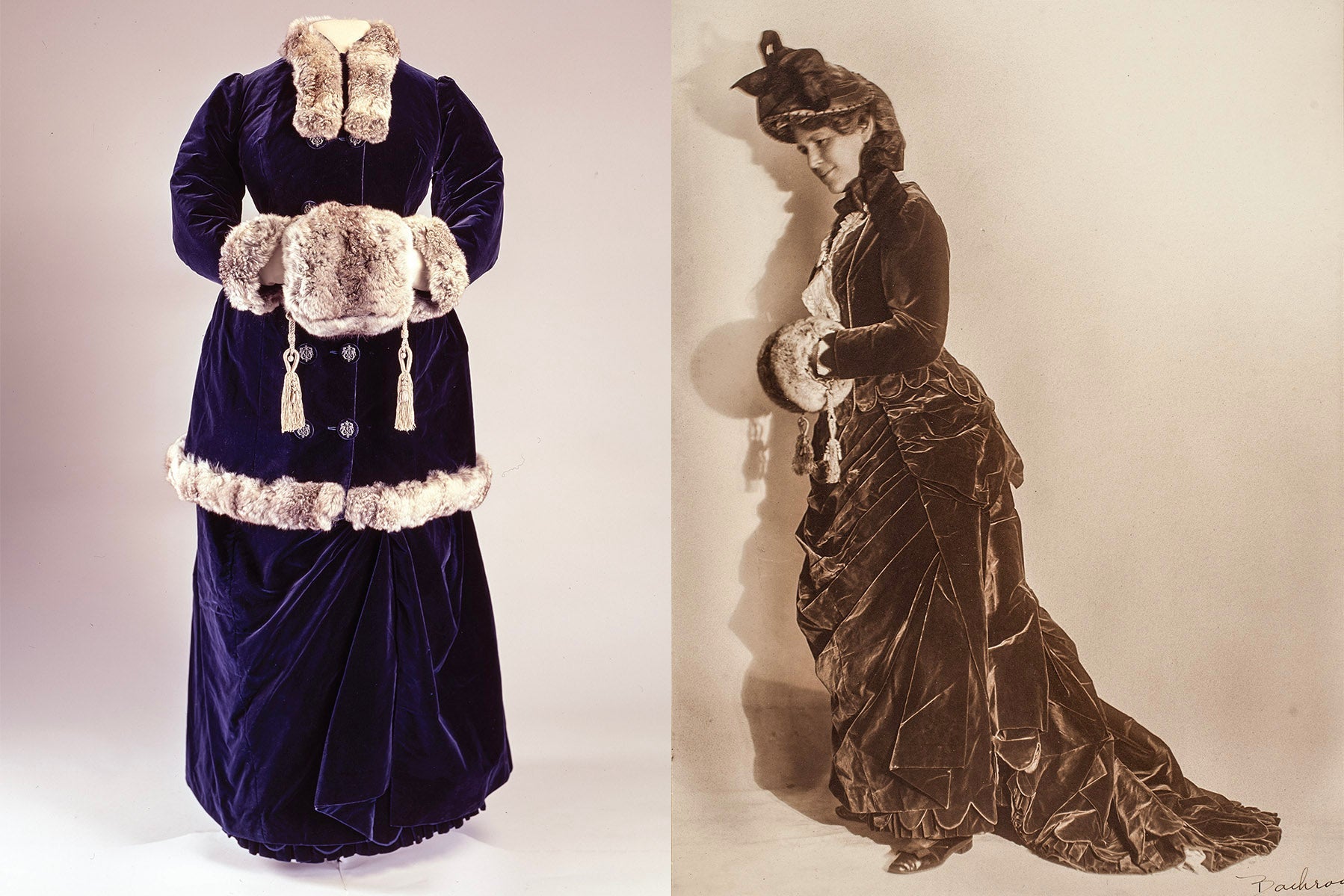The image features a museum exhibit showcasing a royal blue velvet dress ensemble that appears to date back to the 1700s. The outfit includes a double-breasted coat with fur trim on the collar, cuffs, and along the hem, accompanied by a matching fur muff with two white tassels for hand-warming. The exhibit’s dress has a distinctly old-fashioned design suitable for a cold climate, indicated by the extensive use of fur. On the right side of the image, a black-and-white photograph shows a woman from the same historical period, wearing the dress and an elegant hat. Her hairstyle also corresponds to the 1700s, adding authenticity to the depiction. The woman's coat in the photograph is similar, if not identical, to the one in the exhibit, emphasizing the dress’s historical significance. The bottom right corner of the image contains the name "Bachran," adding a point of reference or attribution. The exhibit and photograph together create a vivid portrayal of the dress's intricate design and historical context.